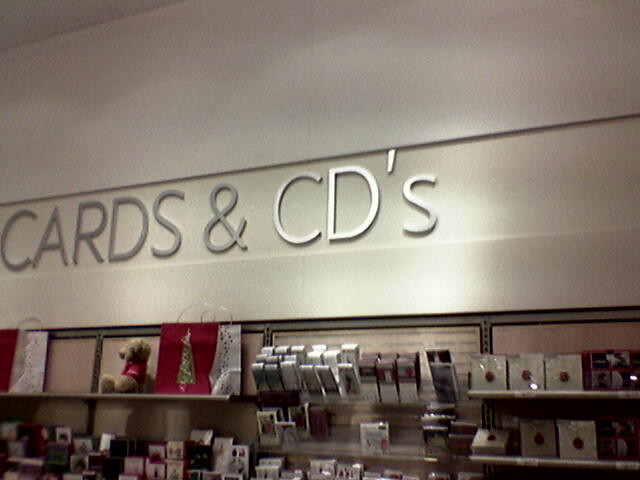The image depicts the inside of a store section labeled "Cards and CD's" with metal, silver, raised letters spanning the wall. The backdrop features brown walls with gray metal dividers and a white upper wall above the merchandise area. The display showcases various cards, although the low resolution makes it challenging to discern specific details. To the right, several cards are wrapped in slightly reflective plastic with a distinctive red dot in the middle, resembling a wax seal. On the left, there's a colorful array of red, green, and white cards, with Christmas-themed gift bags and a stuffed bear in a red shirt positioned on the shelf above them. The decor suggests a festive atmosphere, likely during the Christmas season, accentuated by red highlights and Christmas tree designs on the gift bags. The overall ambiance is somewhat dim, akin to a typical section within a mall-based store.